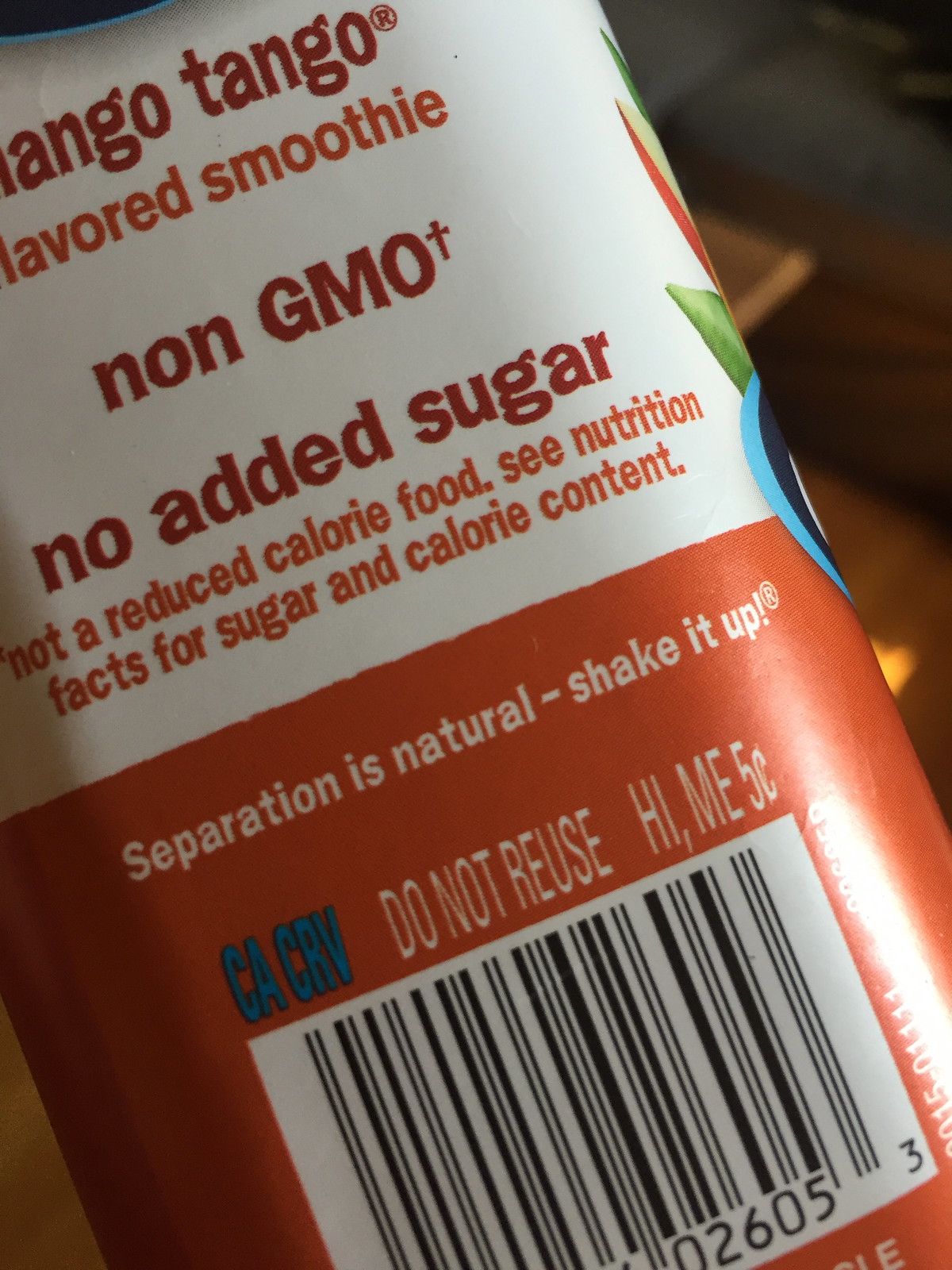This close-up image features the side of a plastic bottle for a "Tango Flavored Smoothie." The bottle is primarily white and dark orange in color, with an intricate label that includes various details about the beverage. Prominently displayed on the white upper portion of the bottle are the phrases "Non-GMO" and "No Added Sugar," followed by the disclaimer "Not a Reduced Calorie Food, See Nutrition Facts for Sugar and Calorie Content." This text is written in dark orange lettering. Toward the bottom, the bottle transitions to a dark orange background with white lettering that reads "Separation is Natural, Shake It Up." Below this, there is a rectangular barcode in a white box, which can be scanned for pricing information. The label also features a visually appealing design with green, red, and blue leaf-like elements. The image background suggests it was taken inside someone's home, as a wood floor and a corner of a table are faintly visible.